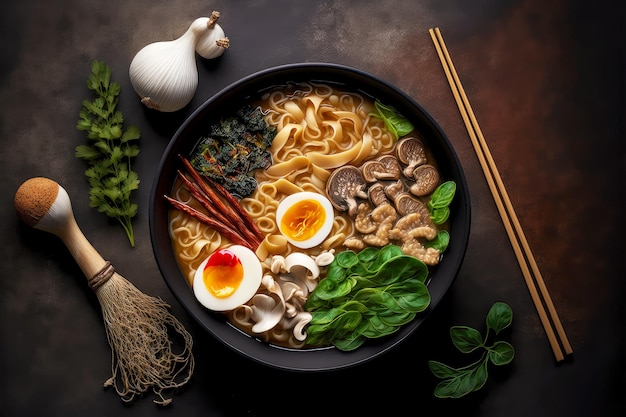The image displays a highly detailed and likely AI-generated representation of an Asian-inspired meal centered in a large black bowl placed on a mottled gray and brown table. The bowl contains an array of vibrant ingredients: prominently, half of a hard-boiled egg with a yellow yolk and a distinct red section sits in the middle. At the 12 o'clock position, there's a portion of pasta noodles, and the 2-3 o'clock area holds mushrooms and additional brown elements. The 5-6 o'clock section features green leafy vegetables, possibly spinach, and there appears to be some white matter, likely chopped onions, at the 6-7 o'clock area. Finally, more noodles and red peppers fill the 8-9 o'clock space, with an unidentified black material at 11 o'clock. Surrounding the bowl, the image includes two bulbs of onions, various vegetables, herbs like coriander, a pair of chopsticks to the right, and some garlic, all enhancing the authenticity of the meal.